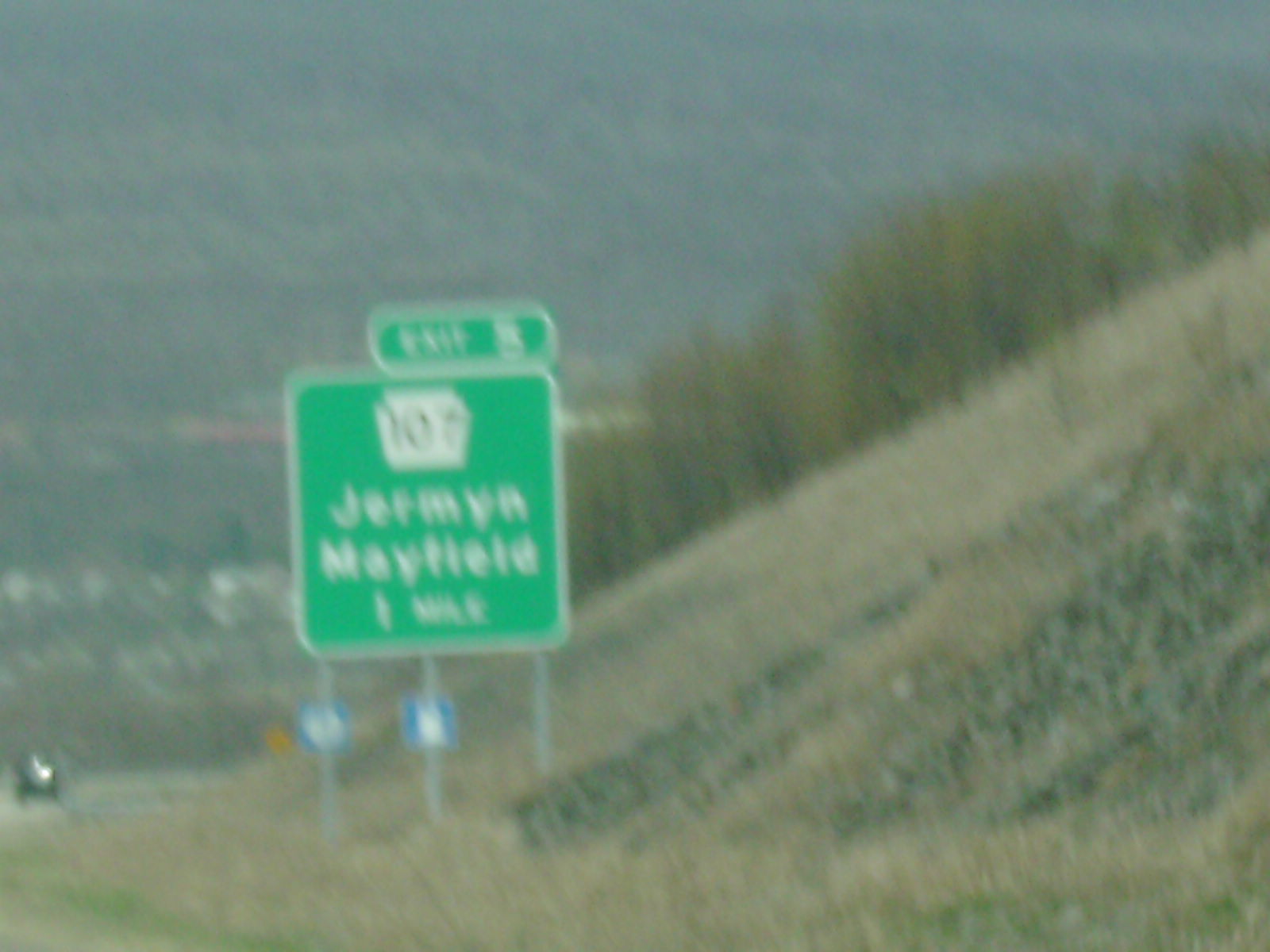This image, taken from the passenger side of a moving vehicle, is slightly blurry and grainy in color, possibly due to motion. The scene depicts a hilly or mountainous area with a prominent slope on the right-hand side, dotted with brown grass, shrubbery, and green trees. In the background, beyond the hill, additional trees cover a large mountain, which is so close that its top is out of the frame. The photo captures a road bending in a semi-circle, with a distant car visible up ahead.

The main focus is a large green highway sign, almost square-shaped, mounted on three steel poles. This sign, bordered in yellow, has white lettering that reads "Exit 5" at the top, followed by "107" and an instruction to reach "German" and "Mayfield," both located one mile away. Below these main directions, there are smaller blue signs, likely indicating services such as fuel, though they are unreadable due to the blur. Towards the bottom of the image, some faraway structures suggest the person's elevated position, offering a view down into a city or town.